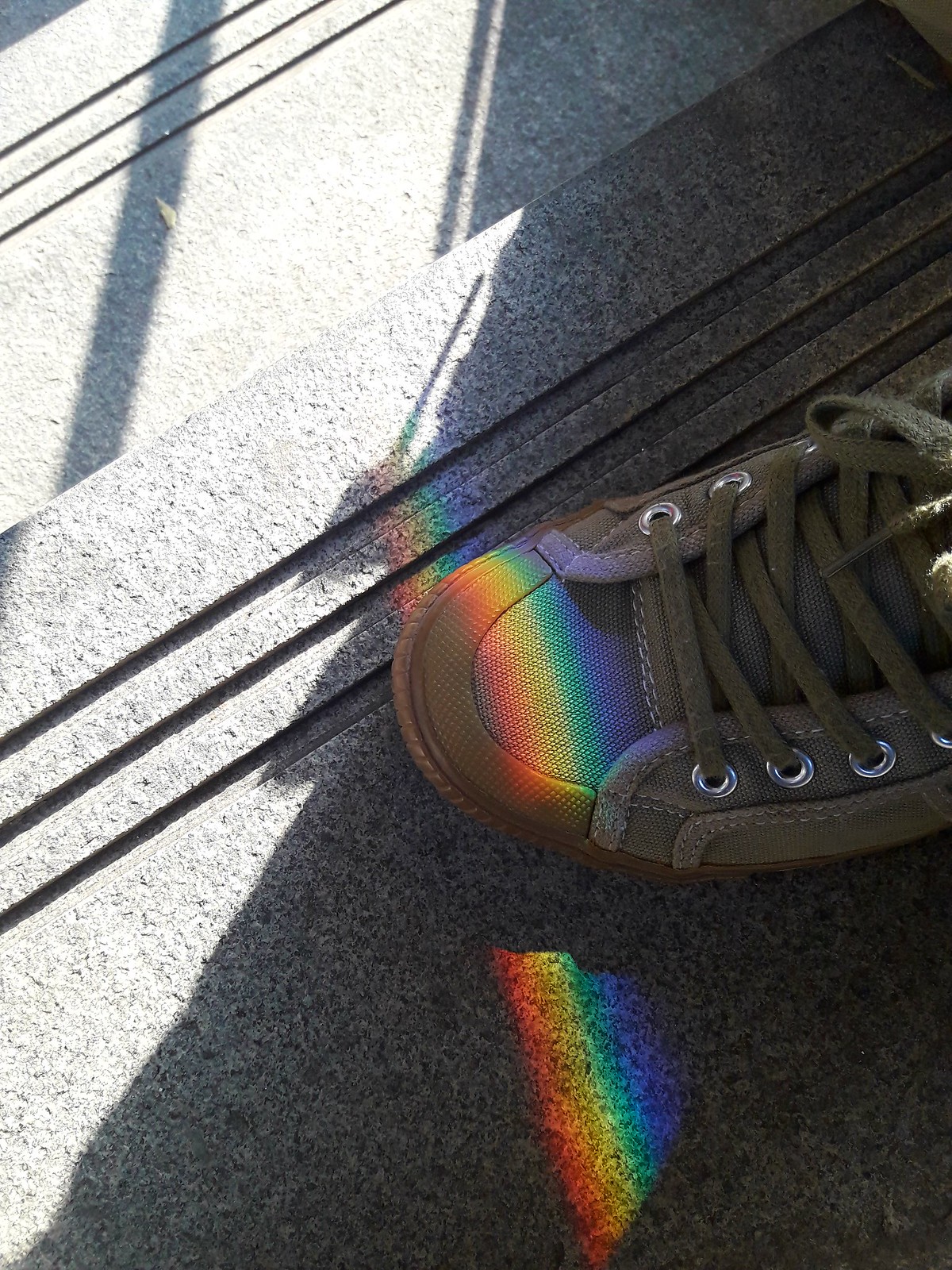A detailed photo captures a single brown shoe with brown laces and silver eyelets placed on a series of grey, granite-like steps featuring diagonal grooves designed for grip. The shoe is positioned towards the right middle of the image, pointed to the left. Sunlight casts a bright reflection, creating a multicolored prism effect over the shoe, transitioning from red to yellow, green, and blue. This daylight shot appears to be taken from above, with the shoe half in shadow and half illuminated, hinting at a boundary between indoors and outdoors. The textured steps and the play of light add depth and interest to the scene.